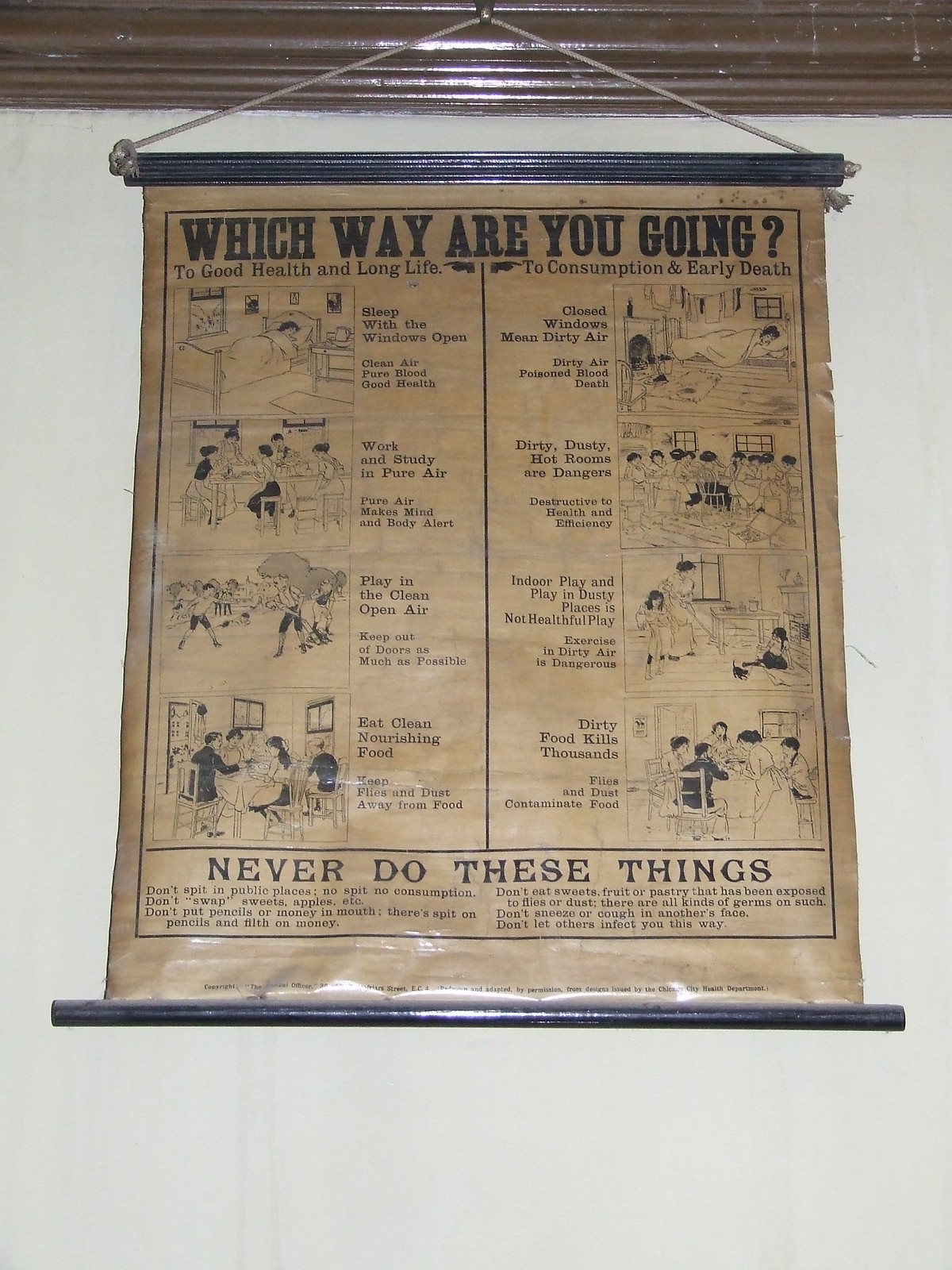This image depicts a vintage health advertisement printed on a brown-aged scroll, suspended from a white wall with brown or dark varnish crown molding. The scroll, which appears laminated and bordered at the top and bottom by black plastic, is centered on the wall and hangs from a rope attached to a nail. The advertisement is structured as a motivating guide, divided into two contrasting paths: one towards good health and long life, and the other towards consumption and early death. At the top, it boldly asks, "Which way are you going?"

The left side promotes healthy habits with illustrations and captions that include a person sleeping with windows open, emphasizing clean air, pure blood, and good health. Other guidance involves working and studying in pure air to keep the mind and body alert, playing outdoors in clean air, and eating nourishing food while keeping flies and dust from food.

Conversely, the right side warns against harmful practices with cautionary illustrations. It mentions that closed windows lead to dirty air and poisoned blood, highlighting the dangers of dirty, dusty, and hot indoor environments. It also advises against indoor play in dusty places and exercise in dirty air, warning that dirty food exposed to flies and dust harbors dangerous germs. Clear instructions label these risks as contributing to early death.

The detailed design of the scroll, with its black and white photographs of people in beds, at tables, and children playing sports, coupled with its vintage typography, enhances the motivational message of health preservation.